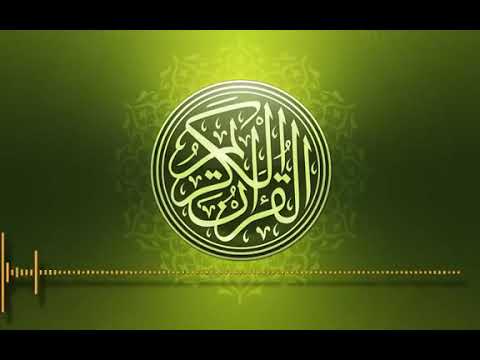This image features a central emblem that appears to be a logo or symbol, surrounded by a detailed and visually intricate design. The emblem consists of three white concentric circles, adorned with a complex arrangement of squiggly lines, small arrows, and various symbols that resemble hieroglyphics or some form of language, possibly Middle Eastern or Asian characters.

The background of the image is a gradient of green, transitioning from dark at the top to lighter in the center, and returning to a dark shade at the bottom. Encircling the outermost white circle is a pattern that resembles leaves and stems, which are in a lighter green color, adding a naturalistic element to the central design.

There are black bars at both the top and bottom of the image, giving it a letterboxed appearance. At the bottom, a series of short, dotted lines runs across the width of the image, resembling an audio equalizer with varying bar lengths, hinting at digital or sound manipulation elements.

The overall orientation of the image is landscape, and the central emblem is prominently positioned in its midst. The intricate design and the detailed elements suggest a symbolic and possibly digital or media-related context.